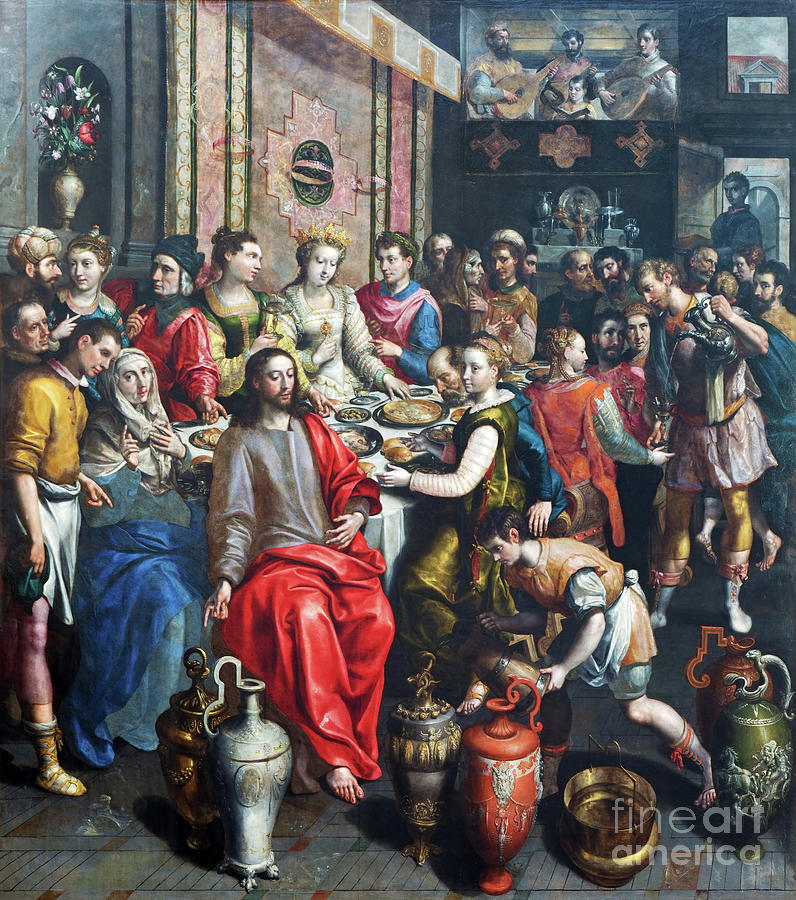The image depicts a detailed painting reminiscent of biblical times, presented in what appears to be a bar or gallery setting. Central to the scene is a large gathering of people, some seated and some standing around a table laden with indistinguishable food on black plates. Many figures are dressed in robes and tunics, indicative of ancient times. A particularly notable figure, potentially Jesus, is positioned at the front, wearing a gray shirt with a long red cloak, while a woman resembling the Virgin Mary in white and blue sits to the left. Surrounding them are individuals adorned in various colors, including yellow, white, gold, red, blue, and multicolored garments. Behind them, the background wall is decorated with flowers in a white vase and features a blend of gold, pink, and red hues. The floor beneath is gray and scattered with an assortment of vases and urns in diverse colors such as gold, white, black, orange, and green. The lower right corner of the image is marked with "Fine Art America." The overall setting impresses as a vivid tableau of a historical feast, rich in color and detail.